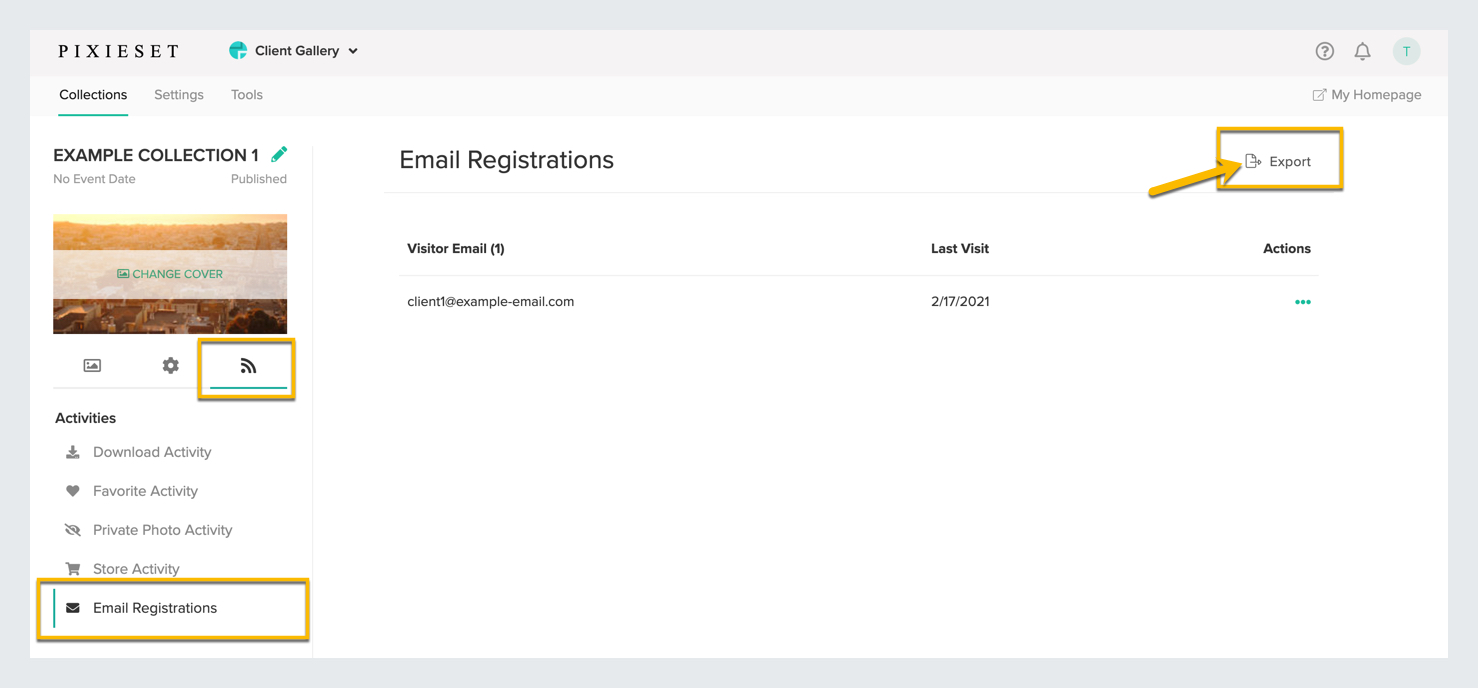This image is a screenshot of the Pixyset software interface. The word "PIXIESET," written in black, all caps, is prominently displayed on a white background. To the right of the Pixyset label, there is a dropdown menu labeled "Client Gallery." Further to the right, there are icons in sequence: a question mark within a circle for help, a bell for notifications, and a "T" possibly representing the user profile.

Directly below this top bar, on the far left, is a navigation menu with the options "Collections" (currently selected and underlined in blue), "Settings" in grey, and "Tools" in grey. The main content area below the navigation menu features a heading: "EXAMPLE COLLECTION 1," accompanied by a blue pencil icon indicating edit functionality. The collection details read "No Event Date" and "Published," alongside a cover image that appears to be an aerial cityscape either at sunrise or sunset; a white banner with the text "Change Cover" in blue overlays this image.

Several buttons are aligned horizontally just below this section. The one resembling a sideways Wi-Fi signal is selected, highlighted by a yellow outline and underlined in blue. To its left is a "Settings" button, and even further left, a "Picture" button.

A series of activity sections are listed below these buttons: "Activities," "Download Activity," "Favorite Activity," "Private Photo Activity," "Store Activity," and, at the bottom, "Email Registrations" which is also highlighted by a yellow outline. This section is expanded to reveal an email registration entry from February 17, 2021 (noted in American date format) labeled "client example email." A yellow arrow points towards the "Export" button, which is similarly surrounded by a yellow outline.